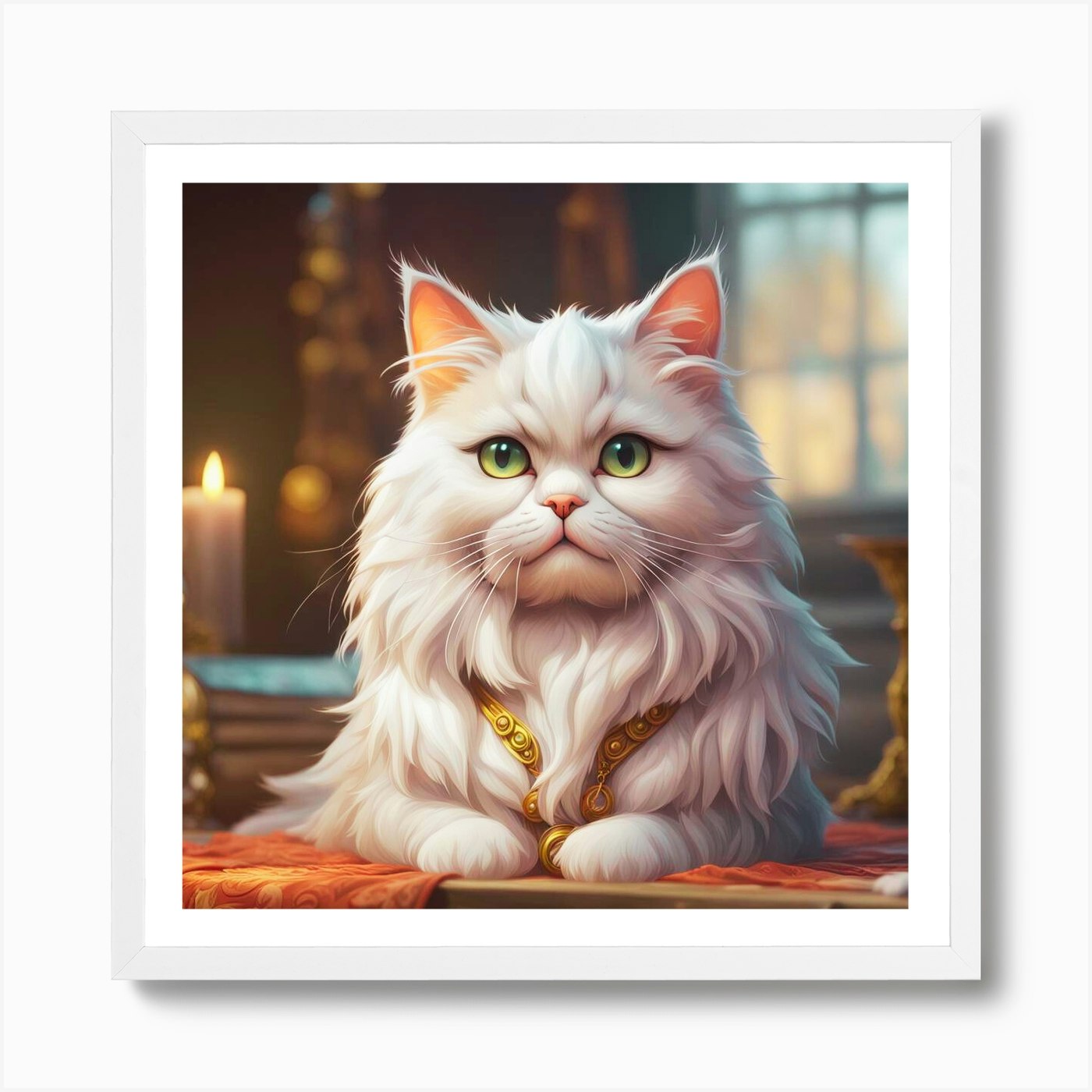In this detailed depiction, a square, animated, or digitally painted photo of a gracefully detailed white cat is enclosed within a white matte and a darker cream-colored wooden frame. The frame casts subtle dark shadows on its right and bottom edges, adding depth to the image. This picture of the cat, which portrays a striking, cartoon-like style, is the focal point and is set against a white canvas backdrop. The feline boasts fluffy, wispy fur, captivating green eyes with black pupils, a distinct pink nose, and long white whiskers. Its erect ears have pink interiors. Adorning its chest is a prominent gold necklace, also styled in an ornate manner. The cat sits on an orange cloth, which adds a vivid splash of color.

In the background, to the upper right, there are blurry, yellowish window panels, possibly hinting at daylight outside. The backdrop features brown walls, and beside the cat is a white candle with an orange flame, adding warmth to the scene. The bottom left of the image incorporates a bright orange and yellow pattern, creating an almost medieval or ornate flair. Together, these elements frame the cat’s serene presence, making the image both vibrant and charming.